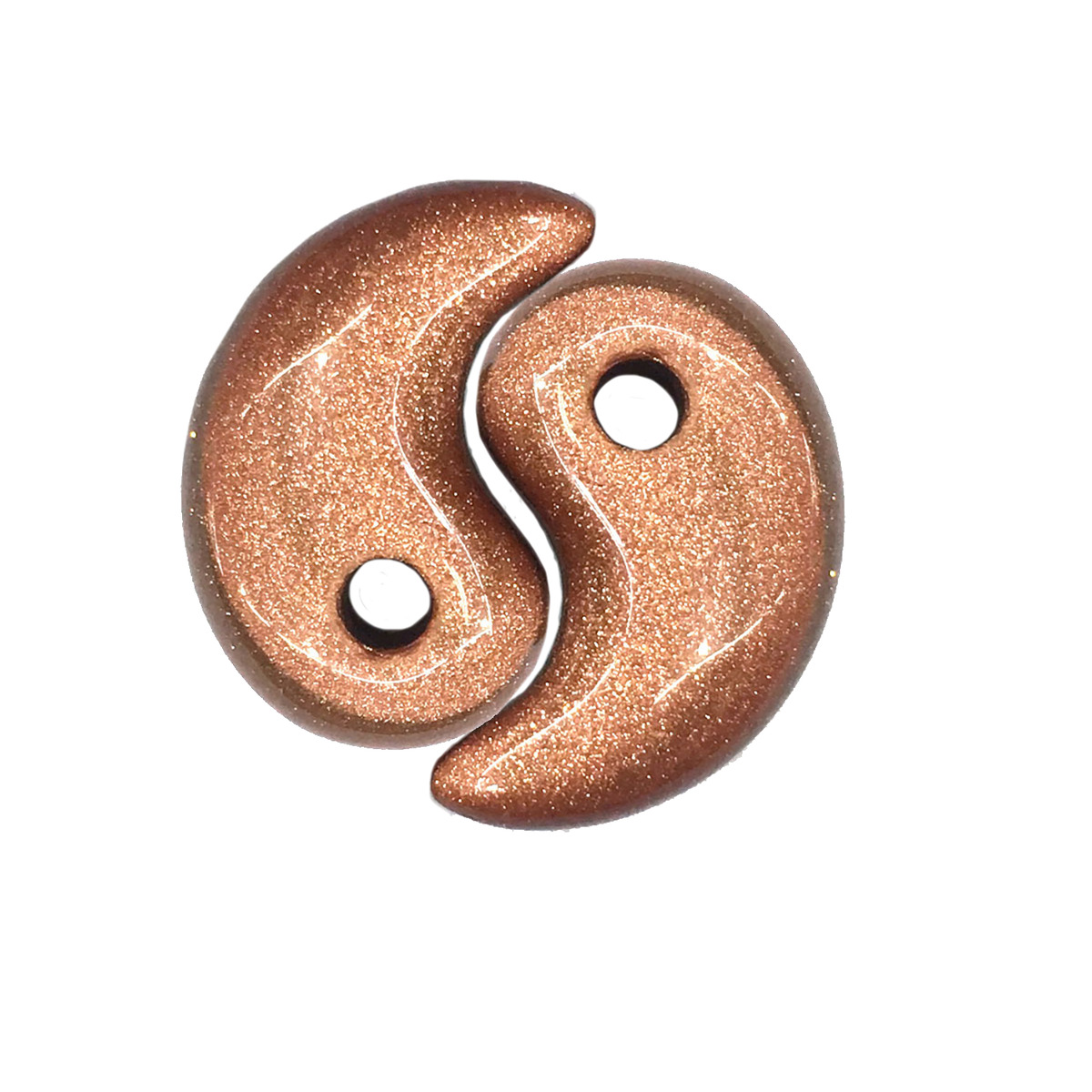The image features two megatama, reminiscent of the yin-yang symbol, positioned at the center against a white backdrop. Each piece exhibits a flowing, teardrop-like curve, tapering off elegantly at the ends and creating a seamless circular shape when joined together. These megatamas are crafted from a copper or bronze-colored material, characterized by a shiny, glittery texture with little white and gold specks throughout, giving them a smooth yet sparkling appearance. Toward the roundish part of each piece, there are holes akin to those found in beads. The polished, artful design suggests that these could be the focus of a product image, potentially for sale on platforms like Etsy.